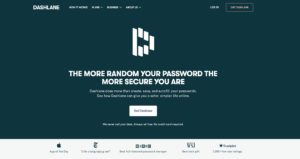The image displays a low-resolution website interface, characterized by its overall poor clarity. In the upper left corner, there is an indistinct word which could possibly be "dash" or "DSL." Adjacent to this are four navigational links. On the opposite, upper-right side, there are two additional navigation links.

Centered prominently on the page is a large, ambiguous icon. Below this icon, a highlighted phrase reads: "The more random your password, the more secure you are." There is smaller, illegible text beneath this phrase. Directly under the icon and text, there is a button containing unreadable text, along with another line of indecipherable text below it. The primary colors used in this section are white text against a dark green background, with the button itself being white.

Further down, the background changes to gray, hosting five more navigation links that are blurred and impossible to read.

The layout of the image is rectangular, with a horizontal orientation. The most prominent text on the page is the adage about password security. Additionally, the logo, located somewhere on the page, is a stylized capital "D" comprised of vertical lines: one for the back, two forming the diagonal stroke, a third outlining the front curve, and two more completing the return stroke to the back.